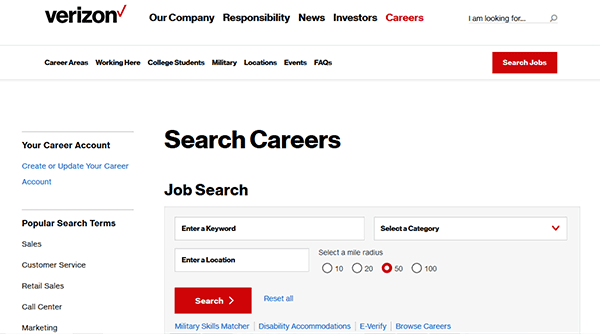This image appears to be a screenshot of a Verizon career page. The upper left-hand corner features the Verizon logo along with the text "BlackTex" and is accompanied by a red check mark. Below this, in black text, there are headers labeled "Our Company," "Responsibility," "News," and "Investors." Adjacent to these headers is the word "Careers" in red text.

On the upper right-hand side, there is a search bar with a prompt saying "I am looking for..." followed by a magnifying glass icon to execute the search. Directly beneath this is another header with various categories in black text: "Career Areas," "Working Here," "College Students," "Military," "Location Events," and "Frequently Asked Questions." Further to the right is a prominent red box with white text that reads "Search Jobs."

To the left-hand side of the page, there are menu headers. The first header says "Your Career Account" in blue text, followed by "Create or Update Your Career Account" also in blue. Below this, in black text, is "Popular Search Terms" with categories listed underneath: "Sales," "Customer Service," "Retail Sales," "Call Center," and "Marketing."

In the main content area of the page, large black text reads "Search Careers." Below it, in smaller black text, it says "Job Search," followed by a series of drop-down menus and text boxes. These options allow the user to enter a keyword, select a category, enter a location, and specify a mile radius with checkboxes available for distances of 10, 20, 50, and 100 miles. In the lower-left corner, there's a red search button with white text labeled "Search." Next to it is a "Reset All" option.

At the bottom of the page, highlighted in blue text, are additional links: "Military Skills Matcher," "Disability Accommodation," "Verification," and "Browse Careers."